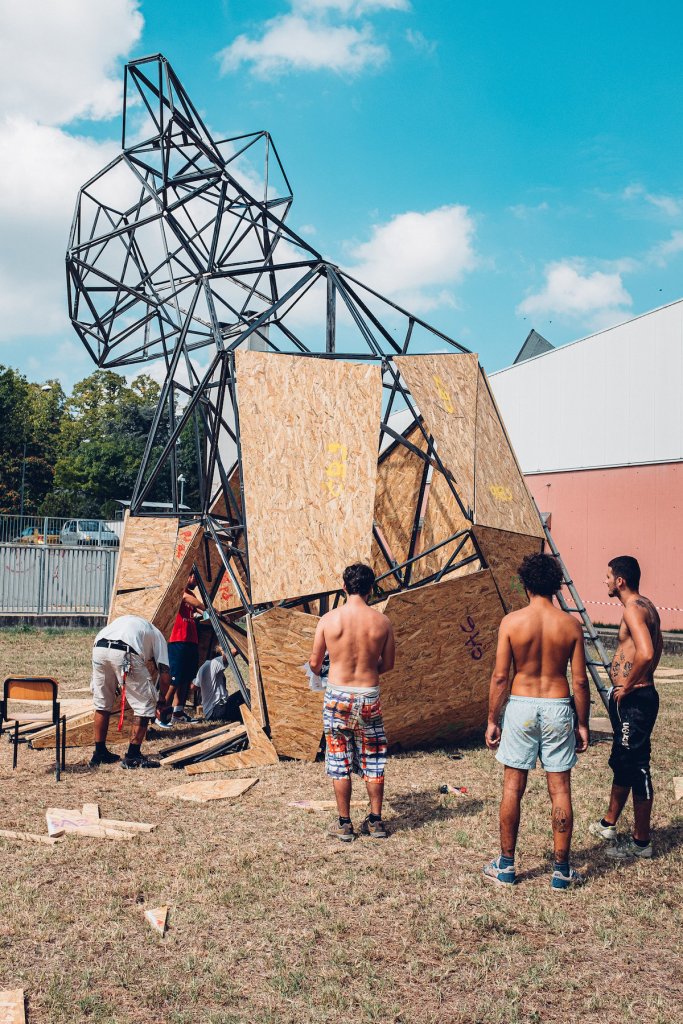In the photograph, five men are diligently working outdoors, assembling a large koala-shaped sculpture. The framework of the sculpture consists of rod sticks being covered meticulously with wooden panels. The setting reveals it’s a hot day under a bright blue sky scattered with puffy clouds. Three of the men are shirtless, wearing shorts; among them, one displays tattoos across his stomach and back, while another shows tattoos on the back of his right leg. A fourth man inside the structure wears a red cut-off shirt, and a fifth man, dressed in khaki shorts and a white shirt, bends over with keys dangling from his belt. They stand on a patch of brown, possibly burnt, grass beside a pink and white building, enclosed by a fence with a parking lot and two cars in the background. Discarded pieces of wood panels and a lone chair are scattered on the grass around them.